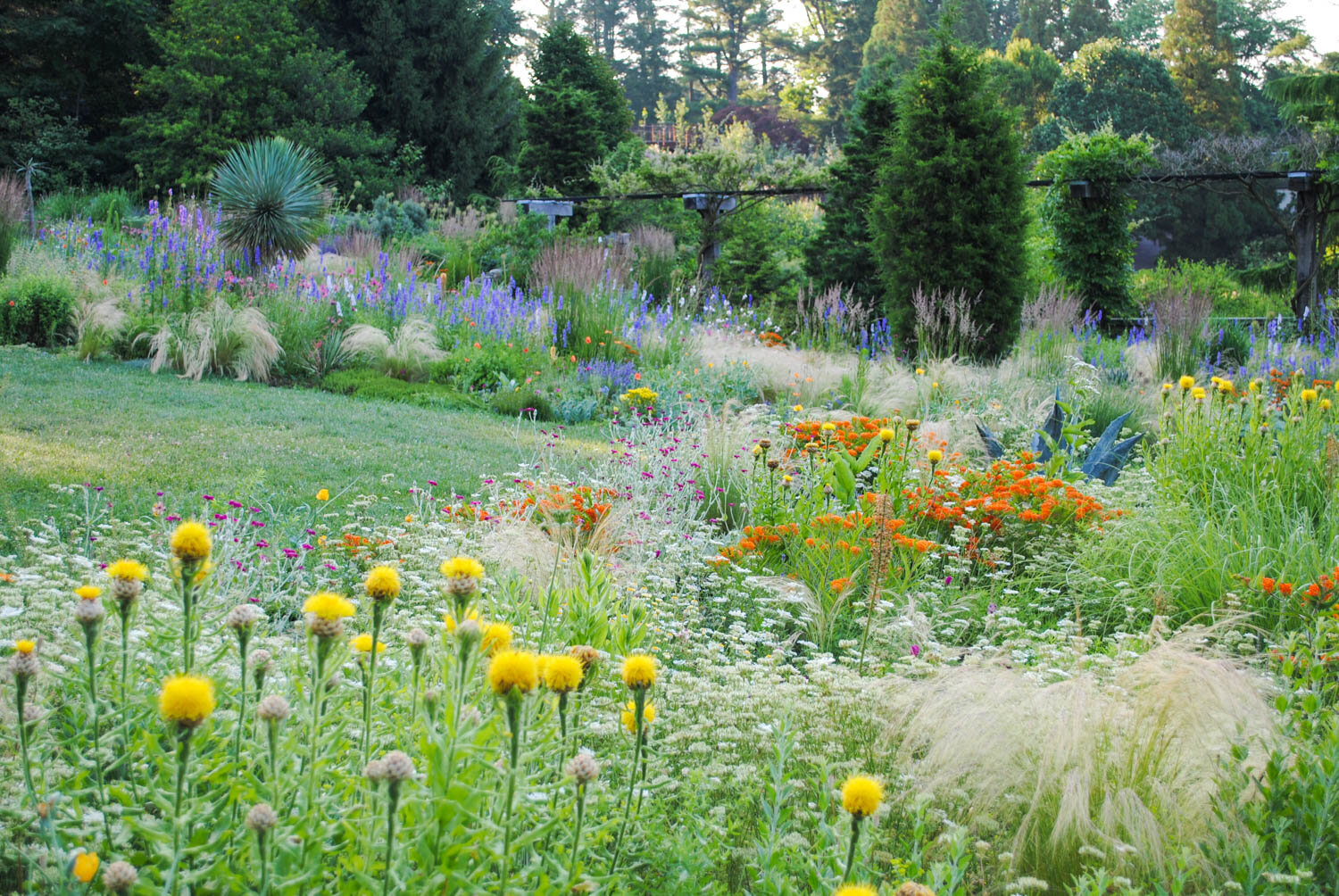This is an outdoor photograph showing a lush, colorful meadow, likely taken in late spring or early summer. The vibrant scene features an array of wildflowers in the foreground with colors ranging from yellow, orange, purple, pink, to white. Among these, some blooms resemble daffodils, and there's also white, wispy pampas grass. The wildflowers grow densely, contributing to the meadow's lively and overgrown appearance.

On the left side of the image, a mowed-down patch of grass seems ideal for a picnic spot, providing a stark contrast to the wildflower-rich areas. In the midground, the meadow transitions into a more grassy area that appears to be a clearing or path, potentially used for walking. 

The background is dominated by a mix of large, full trees, including coniferous varieties like pines, that outline the meadow, suggesting it’s an opening within a forest. Among these trees, there is a structure visible, possibly a metal framework that might be part of a stage or a bridge. Additionally, there are hints of irrigation lines or a fence, implying some human intervention or maintenance. The overall setting is a picturesque blend of wild natural beauty and serene, manicured spaces.